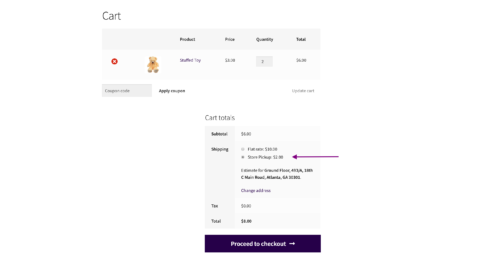This image is a screenshot of a slightly blurry virtual shopping cart, showcasing the summary of the user's purchase as they are about to check out. At the top left corner, one can discern the label "Cart." The main section is divided by headers that categorize the information into columns: "Product," "Price," "Quantity," and "Total." 

Beneath these headers, there is a single row filled out with the details of the intended purchase. The product listed appears to be a stuffed toy, specifically a teddy bear, with a quantity of two. Associated with this product are its individual price and the total cost for the two items. Adjacent to the text information on the left-hand side, there is a small picture of the teddy bear.

Below the product details, a rectangular section offers the option to enter a coupon code, with corresponding buttons to apply the coupon or update the cart, potentially to add or remove items.

In the bottom right section of the screenshot, details of the cart totals are presented, resembling a mini-receipt. Although the screenshot’s blurriness obscures some specifics, the subtotal amount is shown, followed by shipping options: a flat rate or store pickup. The cost for each shipping method is indicated, and a noticeable purple arrow points towards the store pickup option, with the respective bullet point selected, suggesting that this is the recommended or selected choice.

Further down, the total cost, including tax, is calculated and displayed. At the very bottom of the screenshot, a prominent purple button labeled "Proceed to Checkout" invites the user to finalize their purchase.